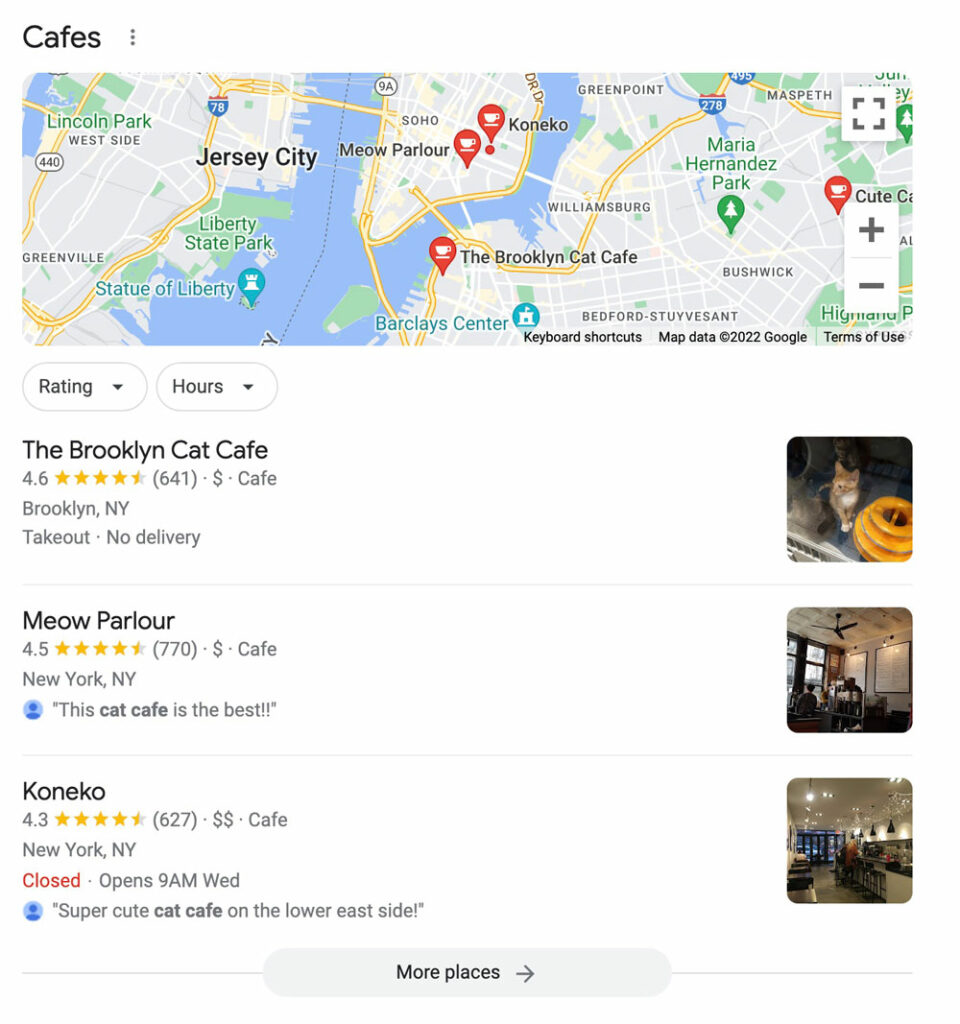This image appears to be a screenshot from Google Maps showcasing a search for cat cafes in the Jersey City and Brooklyn areas. At the top of the screenshot, there are some map icons indicating the search results. The highlighted listings include:

1. **Brooklyn Cat Cafe**: Located in Brooklyn, it boasts a high rating of 4.6 stars.
2. **Meow Parlour**: Another popular option with a commendable rating of 4.5 stars.
3. **Koneko**: This establishment also features prominently, having a rating of 4.3 stars.

In the screenshot, 'Jersey City' is also mentioned, possibly indicating the initial search area. Additionally, the map shows various markers denoting the locations of these cat cafes. Note: There appears to be an unrelated promotional text at the bottom, which reads, "Go to Beadaholique.com for all of your beading supplies needs!"